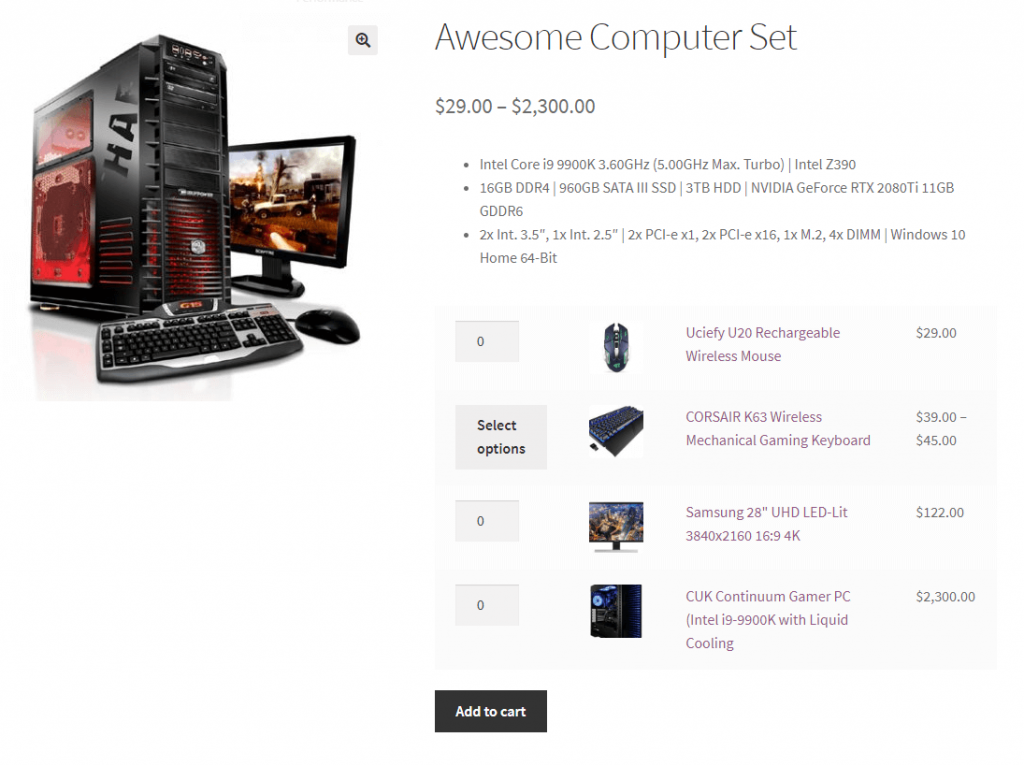The image showcases a detailed view of a high-end desktop computer setup. On the left side of the frame, there is a black desktop computer with a transparent side panel, allowing visibility of its internal components illuminated by red LEDs. The visible components suggest a powerful system designed for gaming or high-performance tasks.

In front of the desktop, there is a black and silver keyboard and a black mouse. The monitor, also black, displays what appears to be a high-end graphics game, suggesting the system's capability to handle intensive gaming applications.

The right side of the image contains descriptive text and images against a primarily white background. The text highlights the specifications of the computer system, advertising it as an "Awesome Computer Set." The price range is listed from $29 to $2,300. A bullet-point list provides detailed specifications:

- Intel Core i9-9900K, 3.6 GHz, 5.0 GHz Max Turbo
- Intel 7390
- 16 GB of DDR4
- 960 GB SATA3 SSD
- 3 TB HDD
- NVIDIA GeForce RTX 1080 Ti 11 GB, GDDR6
- 2 x INT 3.5-inch drive bays
- 1 x INT 2.5-inch drive bay
- 2 x PCIe x1 slots
- 2 x PCIe x16 slots
- 1 x M.2 slot
- 4 x DIMM slots
- Windows 10 Home 64-bit

Additional items listed beneath the specifications include a rechargeable wireless mouse, a wireless mechanical keyboard, a Samsung 28-inch UHD LED monitor, and the Contium Gamer PC. Below these descriptions, there is an "Add to Cart" button, inviting potential buyers to make a purchase.